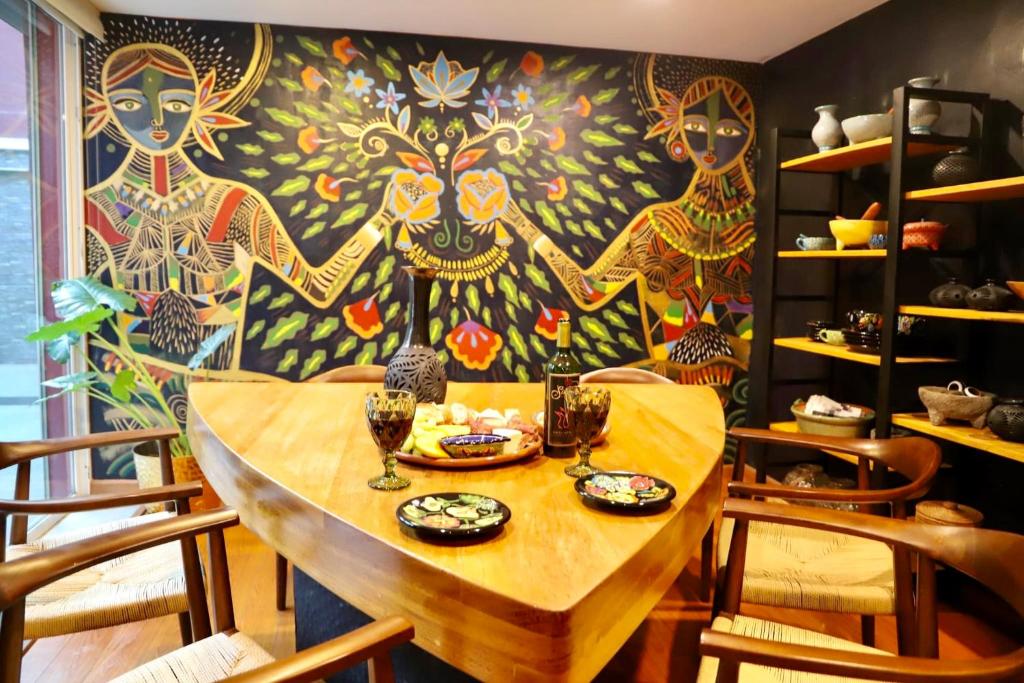This angled interior shot captures a unique and vibrant dining room, possibly in an Indian restaurant. The striking back wall features a large Native American-style mural set against a black background. The mural depicts two vividly colored figures, one on the left and the other on the right, extending their hands towards one another, each holding a yellow heart with a blue outline. Surrounding them is a floral motif with green leaves and various colors including red, orange, gold, and blue, creating a mesmerizing centerpiece that energizes the room. 

In the foreground, a thick, light brown wooden table shaped almost like a triangle stands prominently. On the table, there are two place settings with black plates containing food, an appetizer platter in the center, two goblets filled with a dark liquid, a bottle of wine, and another vase or pouring container. Four wooden chairs with wicker bottoms surround the table, adding to the room’s rustic charm.

To the right, tall black-framed bookcases with yellow shelves are filled with books, trinkets, and various bowls and vases. The left side of the room features a floor-to-ceiling window or door, allowing light to softly illuminate the space. This detailed scene highlights the harmonious blend of cultural artistry and functional design, making the dining room both a feast for the eyes and a welcoming space for a meal.